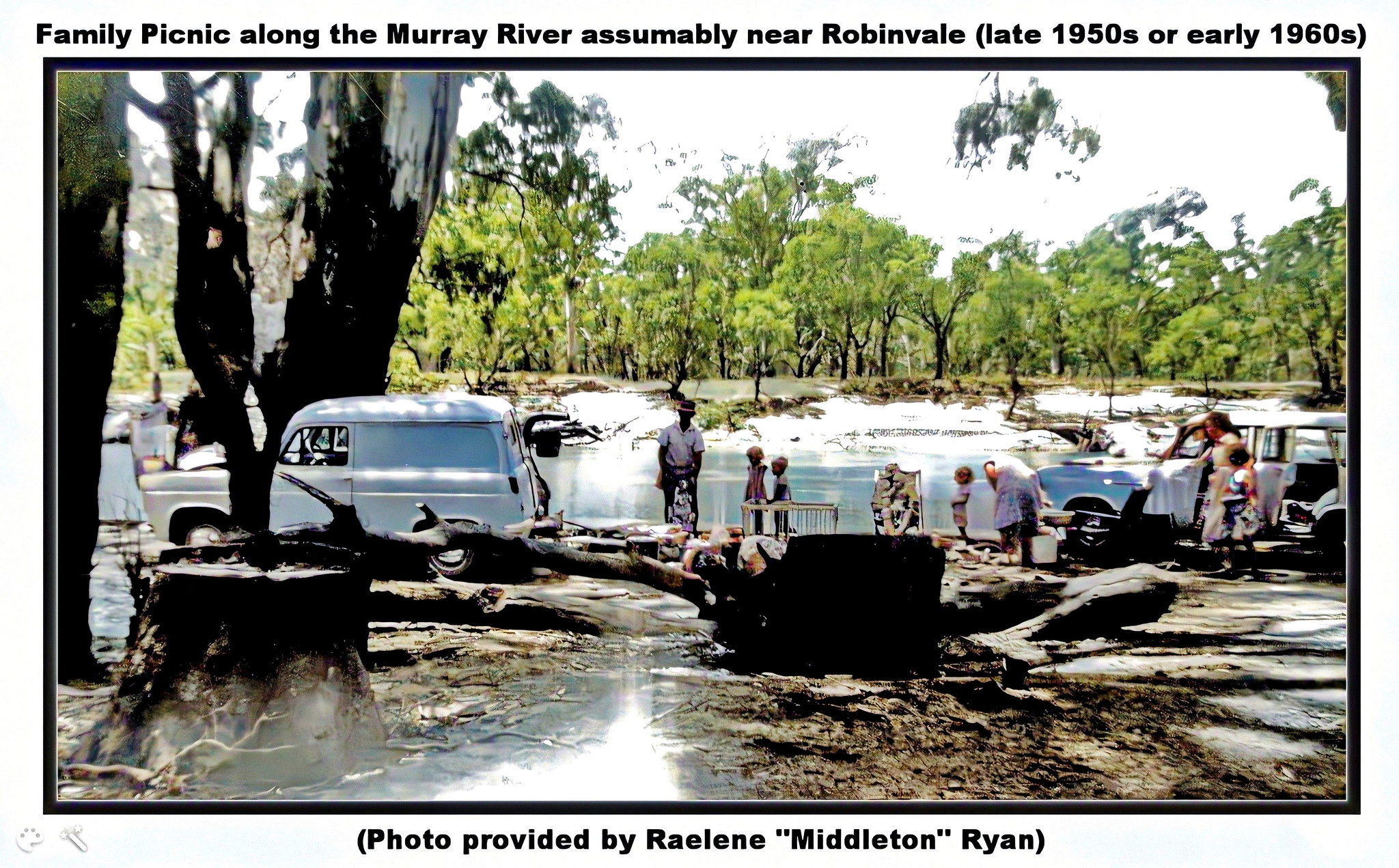This horizontally aligned rectangular picture, bordered in black, captures a nostalgic family picnic along the scenic Murray River, likely near Robinvale, dating back to the late 1950s or early 1960s. Above the border, the text confirms the setting, and below the image, a credit reads, "Photo provided by Raylene 'Middleton' Ryan." The backdrop features a tranquil river with a hint of snow along its bank, framed by rows of tall, leafy green trees under an expansive sky. Along the riverbank, a family enjoys their picnic; two smaller children are safely in a playpen, while others set up chairs and unload items from their vehicles. A white sedan is seen on the left side of the photo, while a white van occupies the right, with people emerging and gathering around. In the foreground, a tree stump and scattered dirt and twigs add a rustic charm to the scene, capturing a slice of leisurely life by the river.